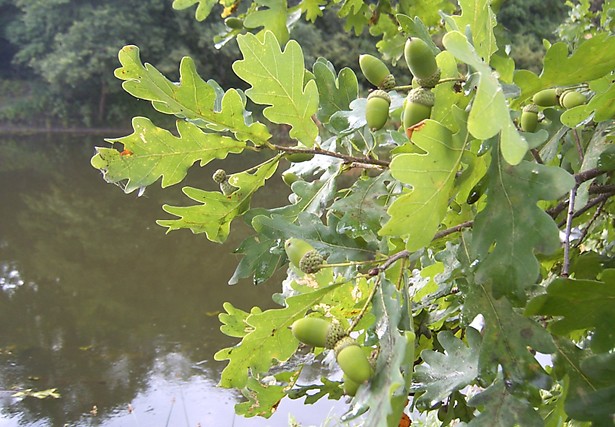The image is a detailed, outdoor, color photograph taken in bright light. The primary subject is a close-up of an oak tree's lower branches, which extend into the frame from the right side. These branches are adorned with large, green, lobed leaves, many exhibiting light green or yellow spots, brown tips, and occasional holes. The branches are heavily laden with an abundance of large, green acorns, each with a rough top and a smooth bottom.

In the background, a calm body of water — possibly a river, creek, or pond — stretches across the scene. The water’s smooth surface reflects the dense, green foliage of the far bank's large trees and thick, bushy vegetation, creating a greenish hue. Additional details include leaves and twigs floating on the water’s surface. The close-up nature of the shot emphasizes the contrast between the detailed textures of the oak tree’s branches and the serene, reflective quality of the water behind them, highlighting the rich, natural environment.